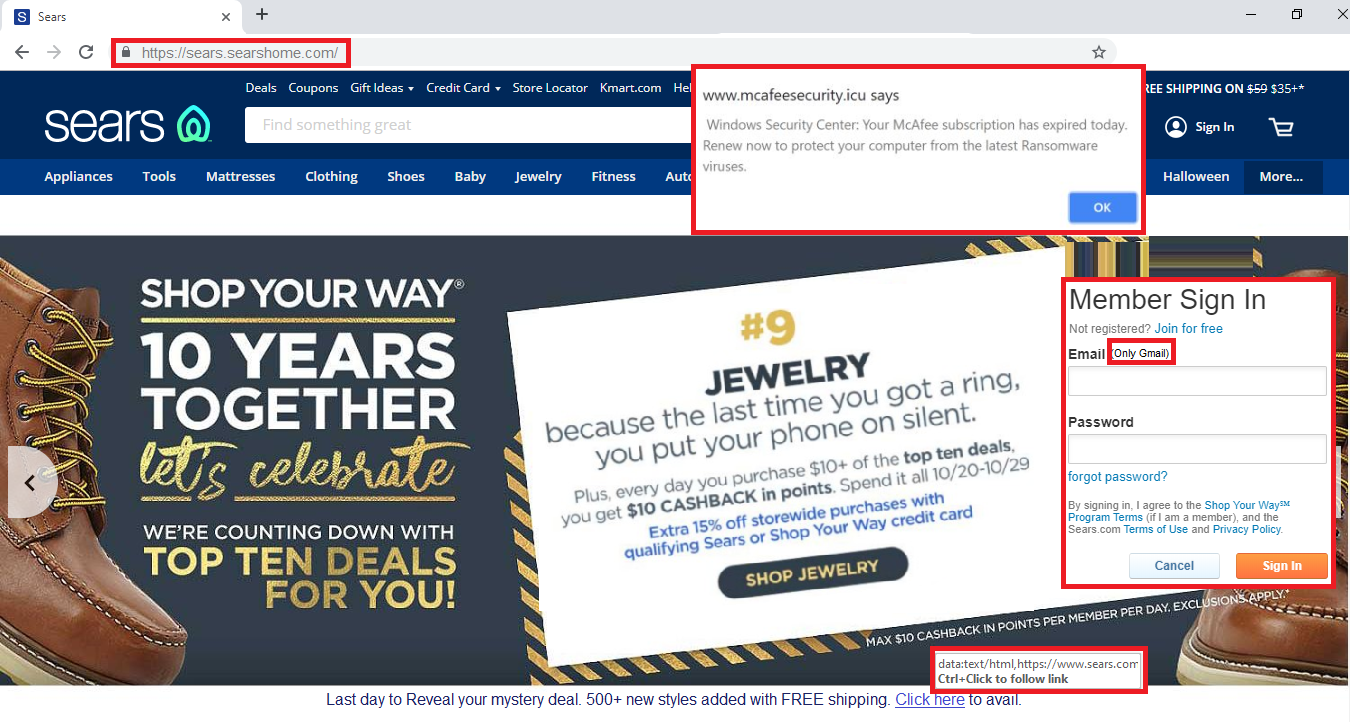The image is a landscape-oriented screenshot of the Sears website, heavily annotated with numerous red markings for emphasis. In the upper-left corner, the browser tab is open, displaying the Sears website (sears.com) as a secure site, highlighted in red. The main navigation bar showcases various categories such as Appliances, Tools, Mattresses, Clothing, Shoes, Baby, Jewelry, Fitness, and Auto.

A white pop-up message, also outlined in red, reads: "McAfee security dot ICU says Windows Security Center: your McAfee subscription has expired today. Renew now to protect your computer from the latest ransomware viruses," accompanied by a blue "OK" button. This unexpected message appears to be part of the screenshot.

Beneath this, an advertisement for "Number Nine Jewelry" is visible, encouraging shopping for jewelry with the tagline, "Because the last time you got a ring, you put your phone on silent." Adjacent to this, there is a sign-in form, also marked in red, with fields for email and password, options for "Forgot Password" and "Join for Free," and buttons labeled "Cancel" and "Sign In."

At the bottom, another red-marked section contains text suggesting navigation details: "Data Text HTML HTTPS www.sears.com control + click to follow link."

This detailed annotation highlights the secure site status, unexpected security alert, promotional and sign-in elements, and technical navigation instructions on the Sears webpage.